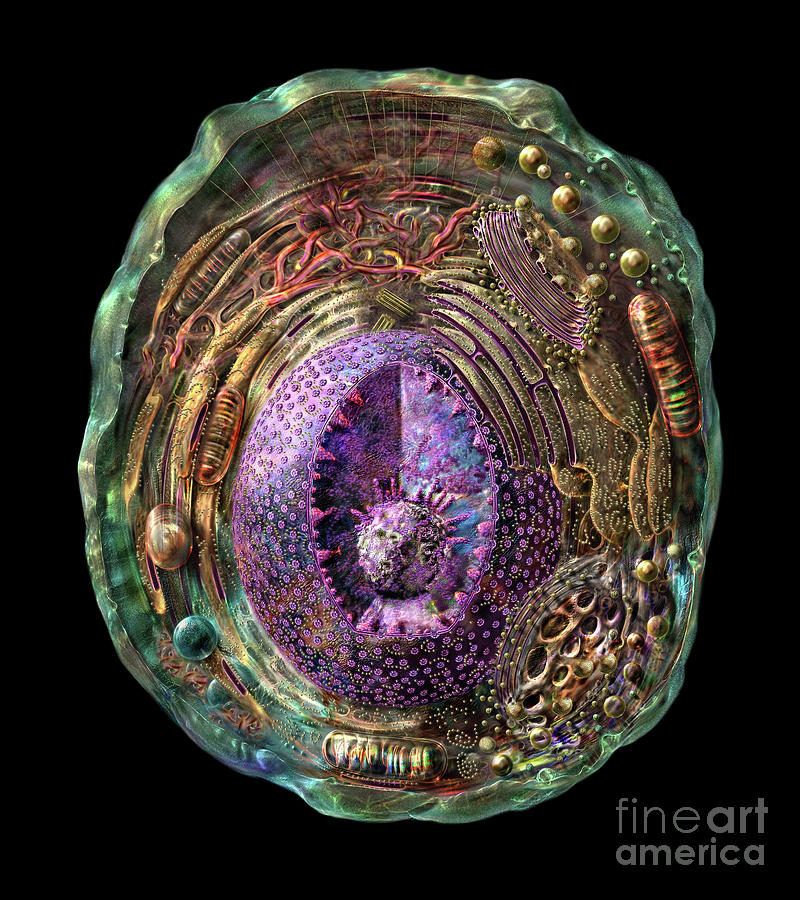This visually striking image, set against a solid black background with a Fine Art America logo in gray at the bottom right, showcases an intricate piece of art that blurs the lines between jewelry and biological illustration. Dominating the frame is an irregularly oval, aquamarine-rimmed structure that evokes the delicate beauty of an abalone shell or a cellular cross-section. At the heart of this artwork is a large, detailed purple nucleus, resembling a sea urchin with numerous purple, dot-like projections. This central feature is surrounded by rings and fragmented arcs of vibrant yellow and gold, interspersed with capsule-shaped, rainbow-colored objects that create a sense of dynamic movement. The image's detailed complexity, with various shapes and multicolored lines, gives an impression reminiscent of microscopic life forms viewed through a high-powered lens, combining scientific intricacy with artistic elegance.